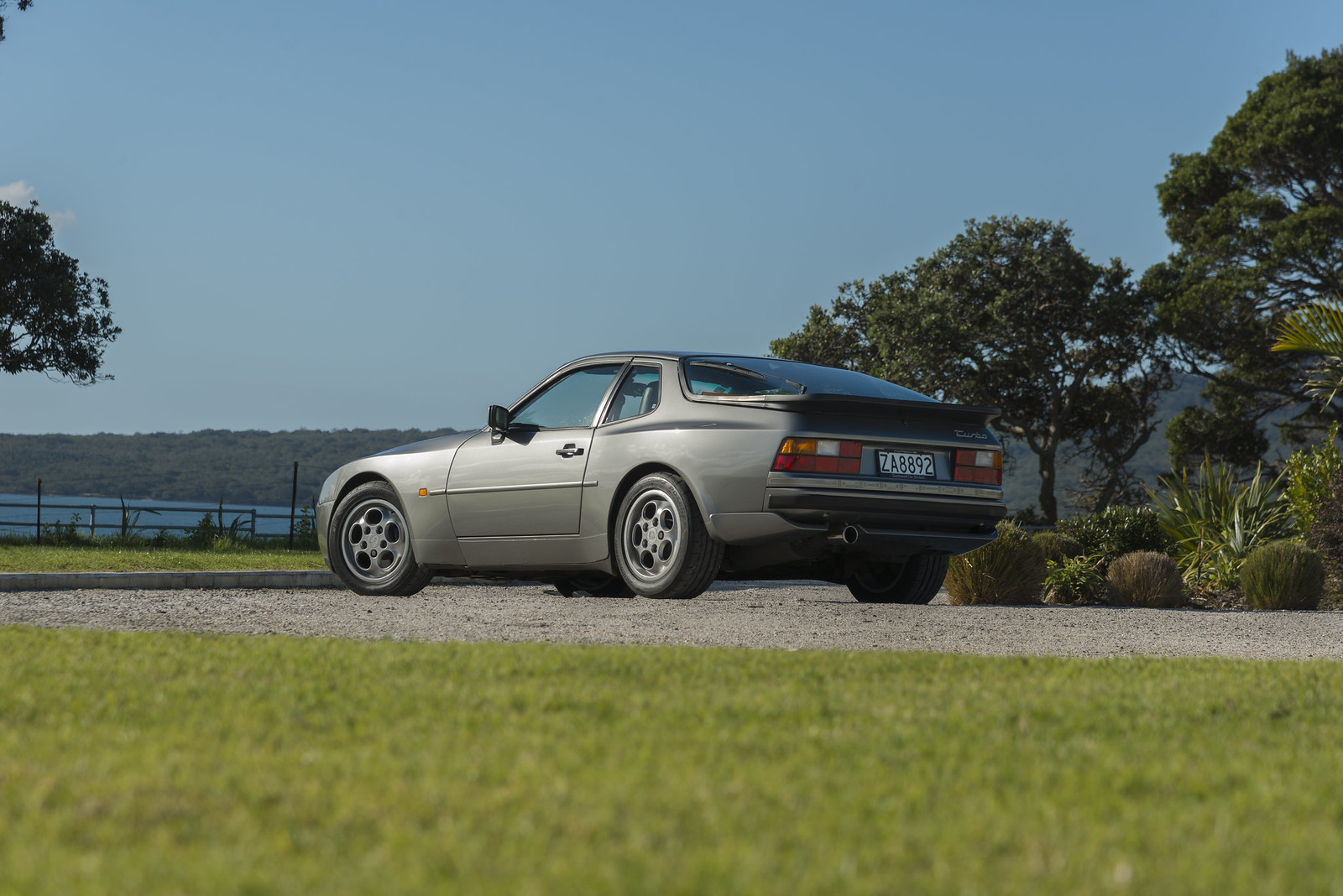The image captures a dated, silver sports car, identified as a 1980s Porsche 944, parked on a gravel road. The vehicle is a two-door hatchback with distinctive features, including metal rims with five drilled holes, a single exhaust pipe on the left, and a rear glass end. Its license plate reads ZA8892. In the background, the serene setting includes a blue sky, a distant large lake bordered by rolling hills, and surrounding greenery with numerous trees and patches of green grass. Additionally, some short shrubs and well-kept landscaping enhance the left side of the scene.